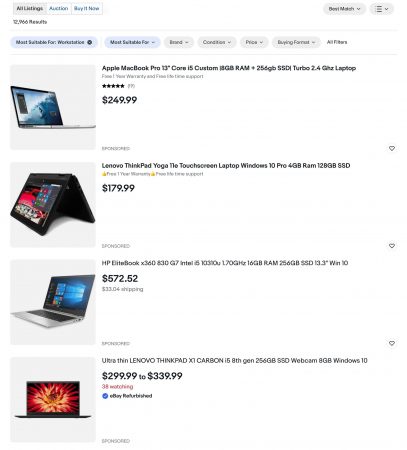A detailed and refined caption for the image could be:

---

A screenshot of an online marketplace, possibly eBay, displaying search results for laptops. The site interface includes a navigation menu on the top left, offering options to view all listings, auctions, and "Buy It Now" items. A search has returned approximately 12,966 results for laptops.

The first visible listing is an Apple MacBook Pro, 13-inch, with an Intel iCore 5 processor, priced at $249.99. Following this is a Lenovo ThinkPad Yoga, featuring a touchscreen and running Windows 10 Pro, available for $179.99. The third item is an HP EliteBook 360, equipped with a G7 Intel processor, priced at $572.52. The last visible listing is the Lenovo ThinkPad X1 Carbon, which is being sold for $299.99. All laptops have accompanying images to the left of their descriptions.

Filters for brand, condition, price, buying format, and more are available to narrow down search results.

---

This caption provides a clear, structured, and detailed description of the image and its contents.